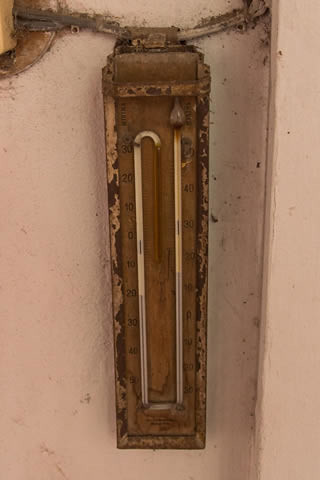In the image, the focus is on an antique device used to measure temperature or air pressure, which appears well-worn and aged. The instrument is predominantly brown, with noticeable areas of rust and degradation. The central part of the device is a darker brown, featuring a long vertical line in the middle that is slightly darker around three inches up. Flanking this line are two white stripes, with numerical markings along both sides. 

On the left side, numbers start at 30 at the top and decrease incrementally, ending at -50 in the bottom left corner. On the right side, the numbers begin at 50 at the top and count down in increments of ten, finishing at -30. The top of the instrument shows substantial rusting and appears to be disintegrating, revealing patches of dark brown paint beneath.

The background features an off-white wall, contributing to the aged ambiance of the scene. Additionally, a long wire runs horizontally just below the top of the instrument, adding further to the antiquated and utilitarian appearance of the setting.